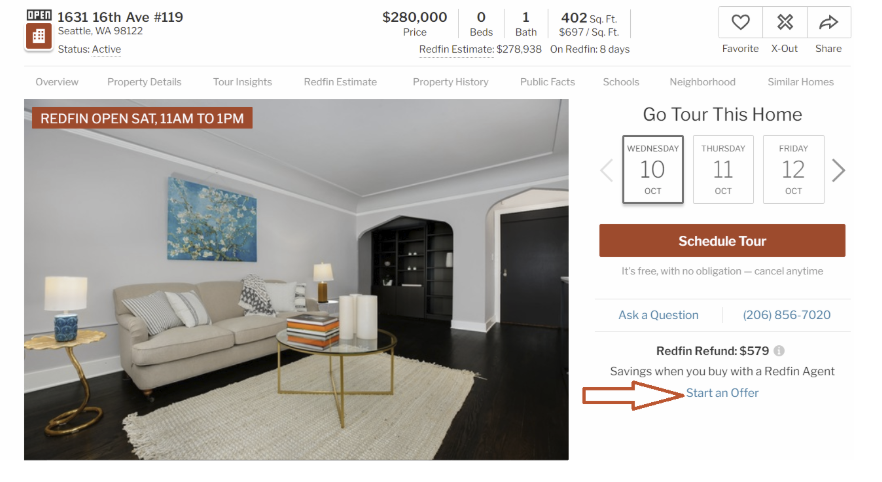Caption: 
Discover this charming studio apartment located at 1631 16th Avenue, Unit 119, in the vibrant city of Seattle, Washington, 98122. Priced at $280,000, this cozy living space offers 402 square feet of modern elegance, featuring an open-concept layout that maximizes the use of space. While the unit boasts no separate bedrooms, it comes equipped with one well-appointed bathroom. The Redfin estimate currently values the property at $278,938 and it has been listed on Redfin for 8 days. Prospective buyers have the opportunity to schedule a tour on either Wednesday, the 10th, or Thursday, the 11th. Don’t miss the chance to explore this exquisite urban dwelling in the heart of Seattle.